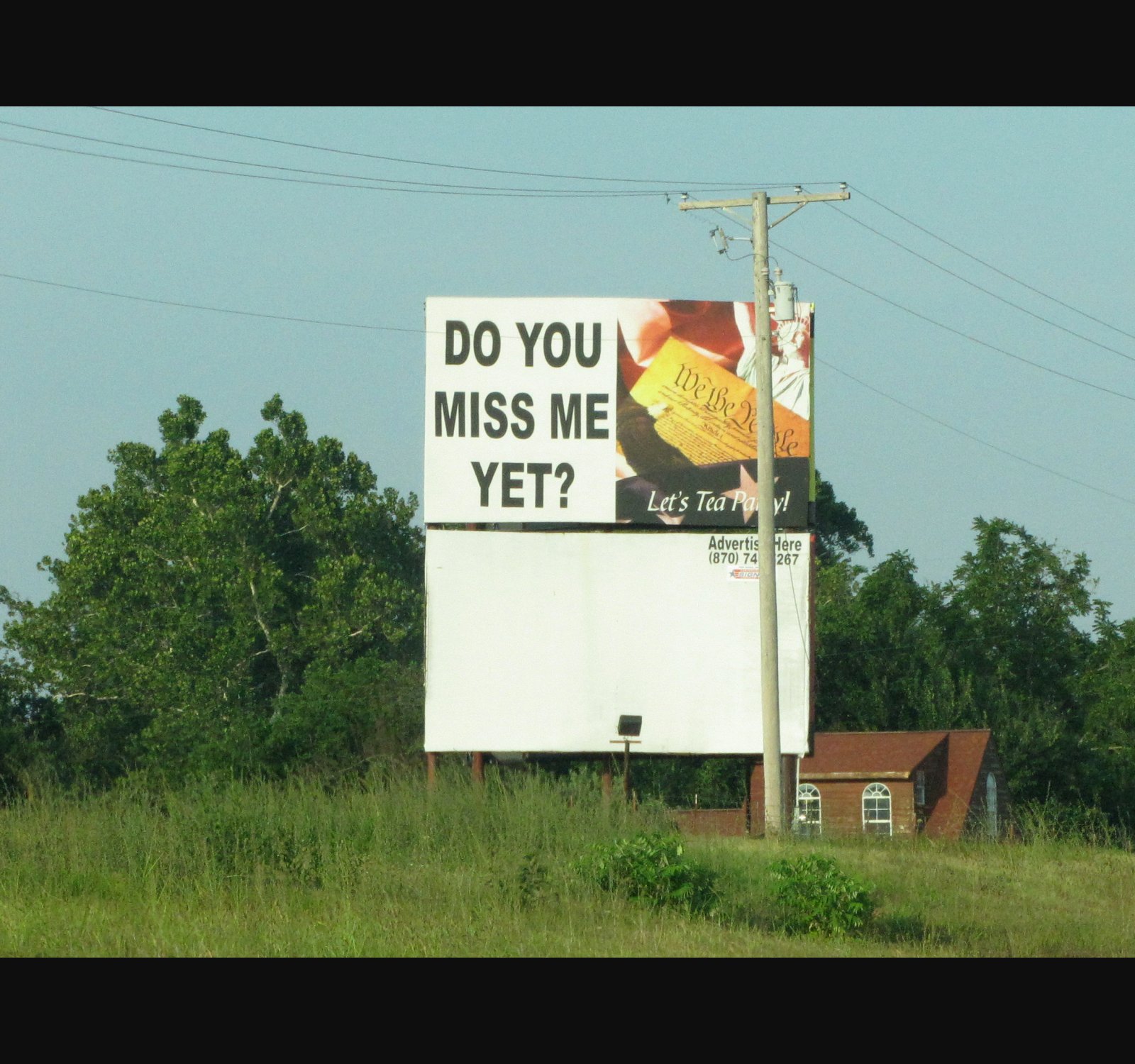The photograph prominently features a large billboard situated at the center of the image. The top part of the billboard bears the text "Do you miss me yet?" written in either black or dark blue on a white background. On the left side of the billboard, the text is paired with a visual element: an image of the Statue of Liberty positioned in the top right corner, and a portion of the U.S. Constitution with the preamble "We the People." Beneath this text, it says, "Let's Tea Party," accompanied by colors reminiscent of the American flag.

Below this main section of the billboard, there is an additional, smaller section that provides information about advertising opportunities, placed against a blank building. The billboard appears partially obscured on the right side by a telephone pole.

In the foreground, lush green grass reaches out towards the billboard, while the background is adorned with trees. Behind and slightly to the right of the billboard, another building is visible, adding depth to the scene. The overall composition blends elements of patriotic imagery with a call to action, set against a backdrop of natural and urban elements.